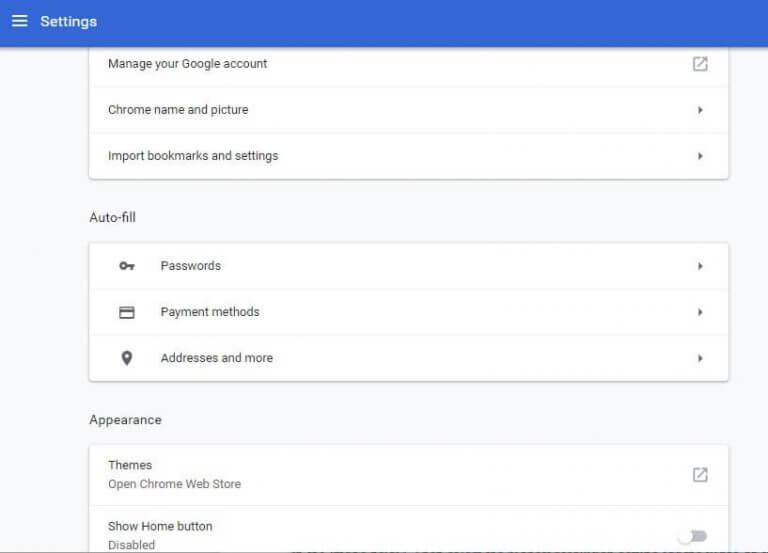The image captures the settings page of a website with intricate details. 

**Top Section:**
On the top left corner, there's a dark blue bezel featuring three horizontal lines, commonly known as a menu icon, used to open the settings menu. Adjacent to it on the right, the word "Settings" is prominently displayed.

**Main Content Area:**
- The background transitions into a light gray shade, adorned with several white rectangular options.

1. **First Rectangular Section:**
   - On the left-hand side of this section, three units are listed in black text:
     - "Manage your Google Account" is the first item. On its right, there's a gray square with a right-facing arrow, indicating a clickable link.
     - "Chrome name and picture" follows on the next line, accompanied by a black arrow pointing to the right.
     - The third line reads "Import bookmarks and settings," also with a corresponding right-facing arrow.
   - Below these options, the text "Autofill" is clearly visible.

2. **Second Rectangular Section:**
   - This section starts with an icon of a key, adjacent to the word "Passwords." On its right, there's another right-facing arrow.
   - Next, an icon resembling a credit card (a square with a line on top, mimicking the back of a credit card) appears next to "Payment Methods," followed by another right-facing arrow.
   - The final item in this section displays a black triangular pin, akin to a Google Maps marker, next to "Addresses and more," also with a right-facing arrow.

**Appearance Section:**
- This part of the settings begins with the title "Appearance" in bold black text.
- The following rectangular option is partially cut off at the bottom:
  - It highlights "Themes" in bold, with "Open Chrome Web Store" below. On the right is a square with an arrow pointing to the right.
  - Underneath this rectangle, within a larger rectangle, there's an option labeled "Show Home Button." On its right, a slider switch is shown, currently in the off position with a white circle to the left, signaling it is disabled.

This detailed description encapsulates the structured layout and various interactive elements present on the website's settings page, offering a clear visual guide.